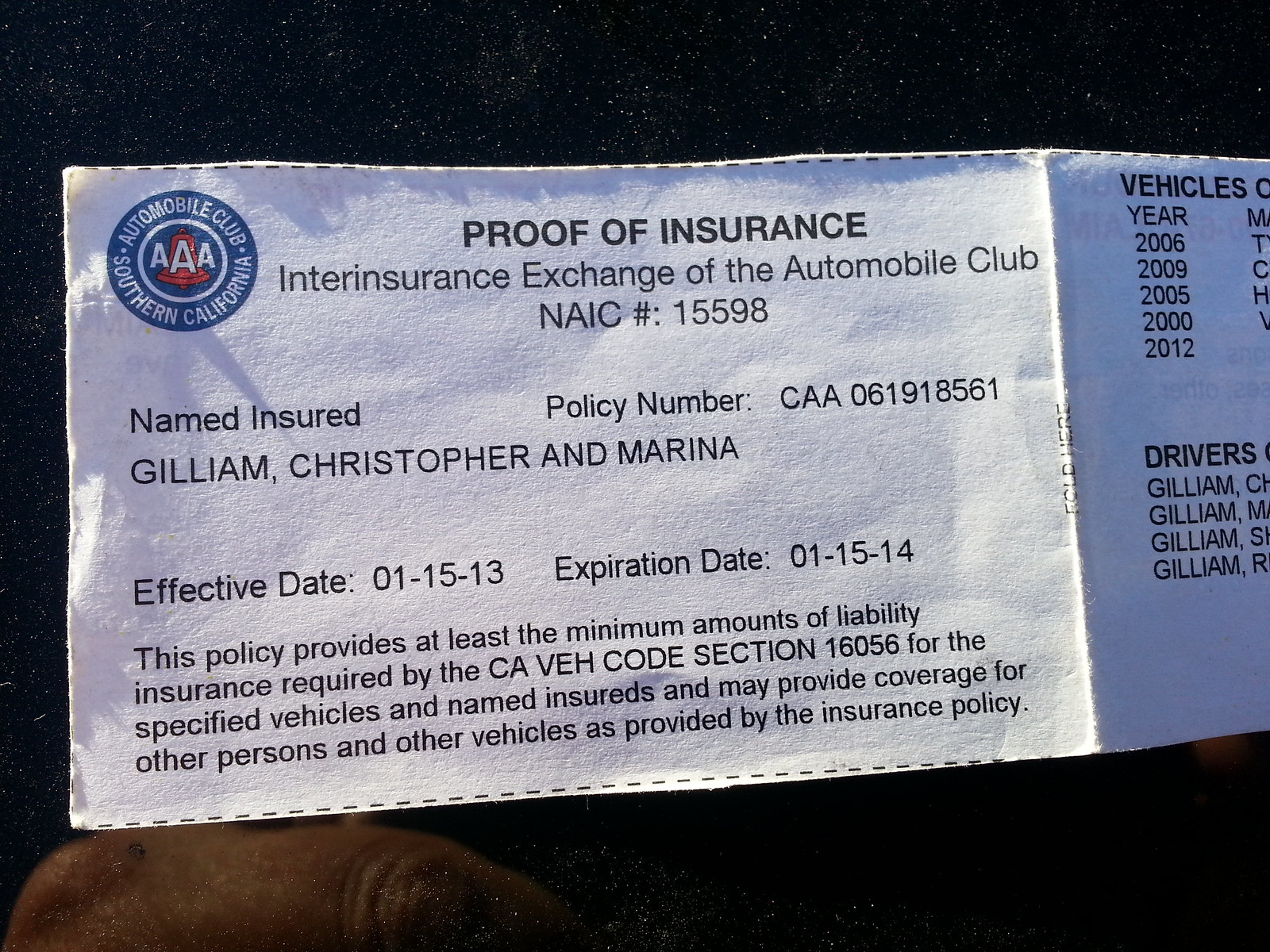This image captures a close-up photograph of an unlaminated proof of insurance document for the Southern California Automobile Club. The document is a non-rectangular piece of paper, folded and creased in the middle, suggesting it was intended to be cut along the dotted lines around its edges.

The left section of the document prominently displays the AAA seal in the upper left corner, with "Proof of Insurance" across the top. This section contains personal information, including the names of the insured, Christopher and Marina Gilliam, as well as the policy number. The effective date of the policy is January 15, 2013, with an expiration date of January 15, 2014. Below this are four lines of printed text, explaining that the policy meets the minimum liability insurance requirements per California Vehicle Code sections and may cover additional persons and vehicles as detailed in the policy.

To the right of the crease, although partially cut off by the image's edge, the document lists details under headings "Vehicles" and "Drivers." The visible entries detail vehicle years such as 2005, 2009, and 2012, but not specific car models. The driver's section shows the last names of the individuals covered under the policy but only partially reveals their first names. In the bottom left corner of the image, a portion of a person's hand is visible underneath the paper, indicating it is being held up against a flat surface, perhaps the windshield of a car.